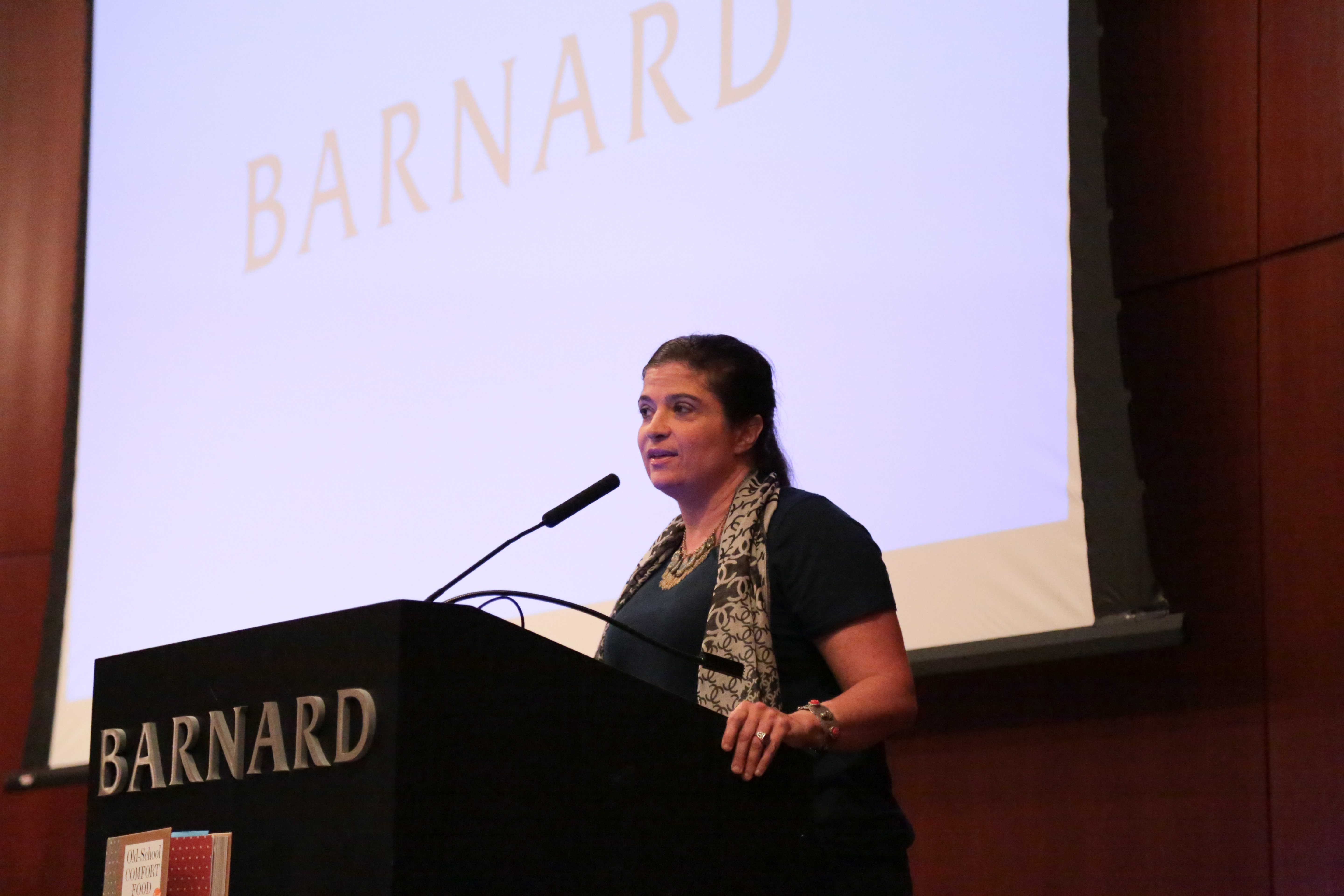In the image, a woman is standing behind a black podium, delivering a speech into a black microphone. On the front of the podium, raised grey letters spell out "Barnard." The background features a brown wooden wall composed of varied pieces, and a white projector screen is pulled down, also displaying the word "Barnard" in red text. The image is slightly tilted, with the viewer positioned to the speaker's left. The woman has olive-colored skin and long dark hair pulled back. She is wearing a black short-sleeve shirt and a patterned scarf that features shades of brown and beige. A silver ring adorns her hand, and she has a bracelet on her wrist. The left side of her body is more visible, emphasizing her accessorized arm as she grasps the podium.